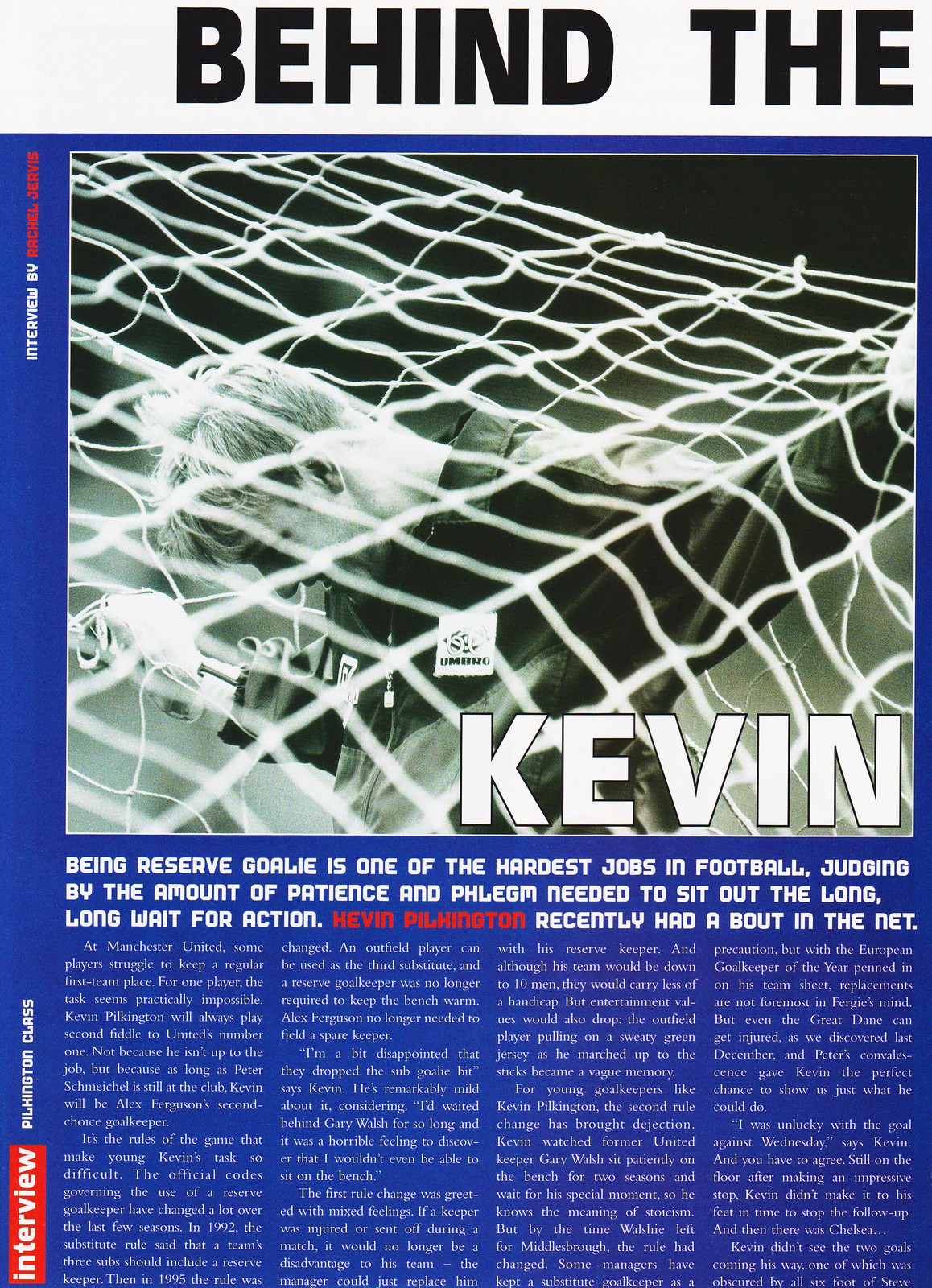The image is a detailed scan of a magazine page featuring an article titled "Behind the Kevin." The page, primarily in blue, includes various text colors such as white and red that highlights certain words. The majority of the layout is occupied by a striking black and white photograph of a man, Kevin Pilkington, tangled in a soccer net. Pilkington's figure is central in the image, with his head bowed forward and the net enveloping him, creating a sense of struggle and entanglement. This intriguing centerpiece is situated above several columns of text that delve into Pilkington's experiences and challenges as a reserve goalie in football. The article header "Behind The" is prominently displayed at the top, while the name "Kevin" is placed in bold text at the bottom right corner of the image. Overall, the page vividly portrays the patience and resilience required in Pilkington's demanding role.